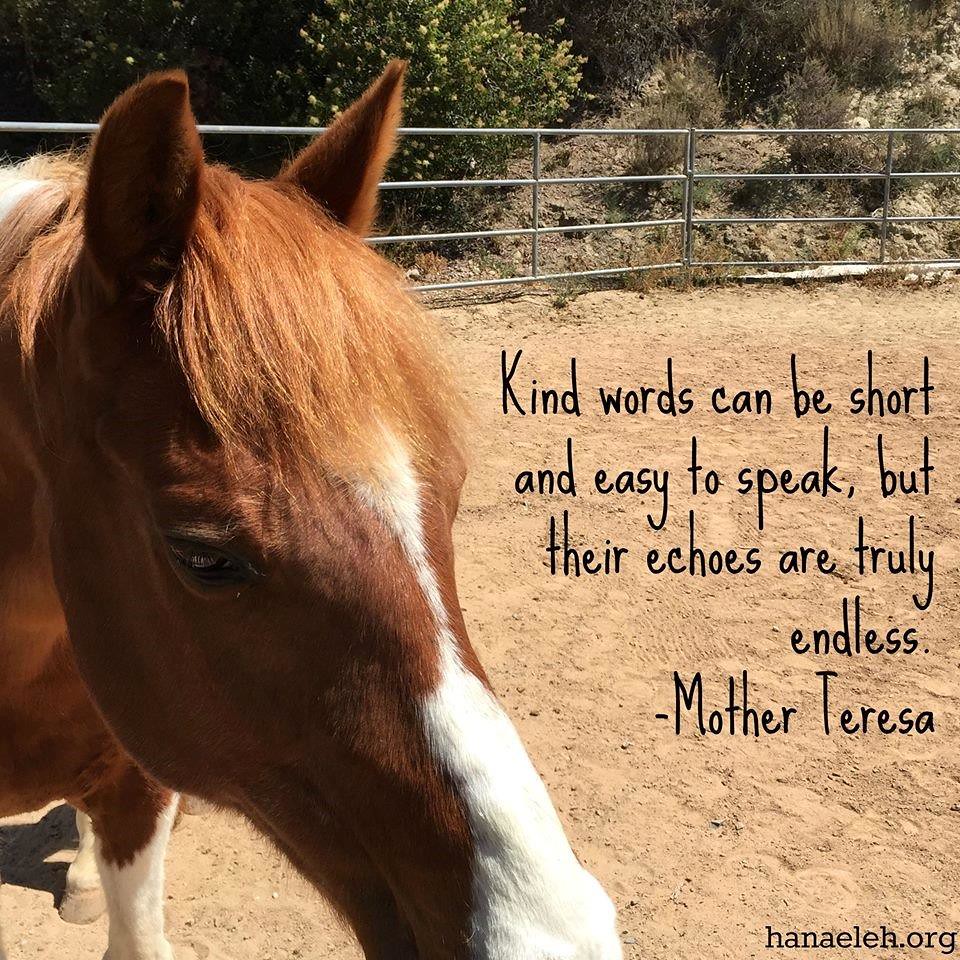This square image, potentially a poster or a note card, features a close-up photograph of a young brown horse with a noticeable white stripe running down its nose. The horse, positioned on the left side of the image, gazes directly at the camera, its reddish-brown mane partially covering its eyes. Its white-bottomed legs transition to brown at the top, complementing its brown, upright ears. The scene captures the horse standing in a dirt field enclosed by a metal fence that forms a corral, with a backdrop of bushes and a hillside. On the right side of the image, a quote by Mother Teresa is elegantly inscribed in a fancy font: "Kind words can be short and easy to speak, but their echoes are truly endless." Below this quote, the website "Hanaeleh.org" is noted in smaller black letters.